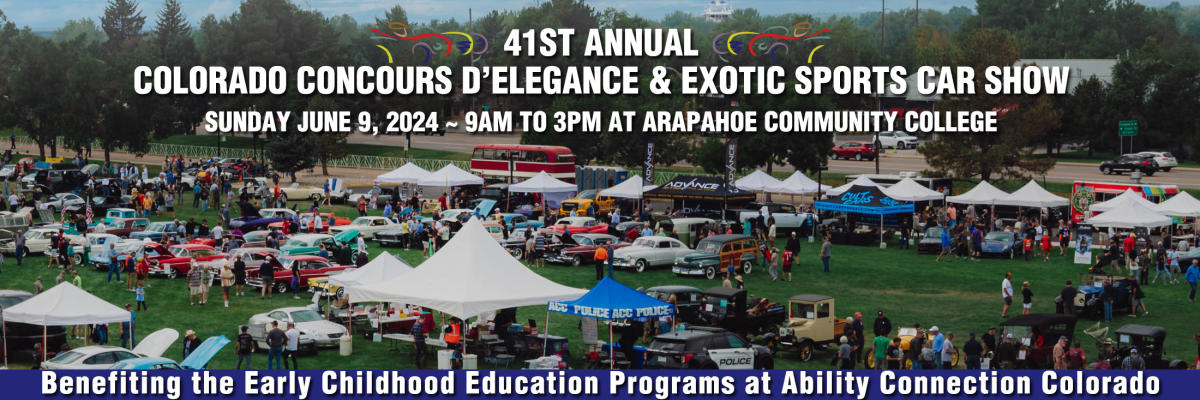The banner image advertising the 41st Annual Colorado Concours d'Elegance, an exotic sports car show, features bold white lettering at the top, stating: "41st Annual Colorado Concours d'Elegance, an exotic sports car show, Sunday, June 9, 2024, 9 a.m. to 3 p.m. at Arapahoe Community College." Additional information at the bottom, also in white text bordered in blue, reads: "Benefiting the Early Childhood Education Programs at Ability Connection Colorado." The central photograph, captured from an aerial view, showcases a bustling car show on a verdant, grassy expanse. Numerous vintage and muscle cars, including a woody station wagon and colorful old-time automobiles, are meticulously arranged in rows. Crowds of spectators meander among the cars, under tents and awnings interspersed throughout the fairground. Vendors and exhibitors add to the lively atmosphere, with a double-decker vintage bus standing out. Green trees border the area, contributing to the picturesque park-like setting. This stunning and detailed photograph encapsulates the vibrant spirit of the event, enhancing the promotional banner.